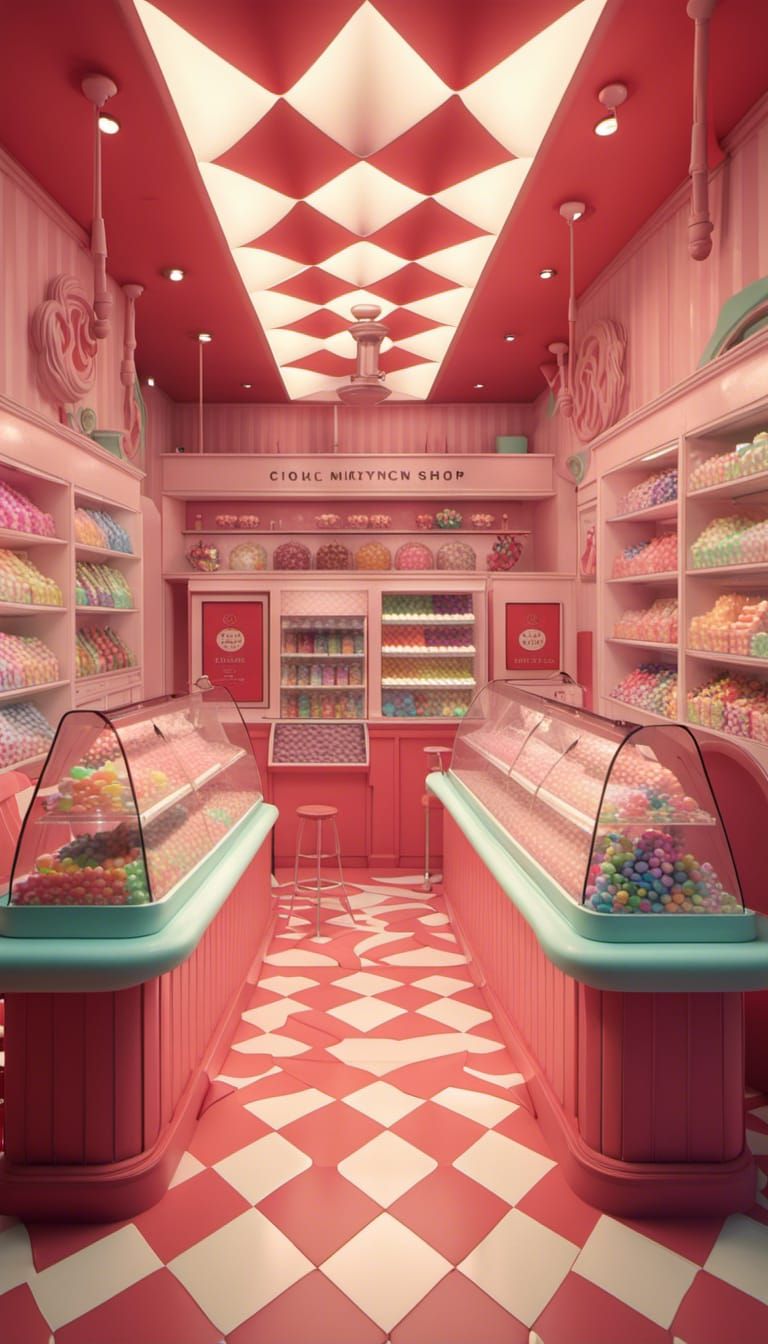This digital art rendition, possibly AI-generated, depicts a charming and somewhat realistic candy store. The narrow room is predominantly decorated in shades of pink and white, creating a whimsical atmosphere. The floor features a pink and white diamond-checkered pattern, while the ceiling showcases alternating pink and white stripes with recessed and hanging lights that add a warm glow.

The shop's walls are adorned with light and dark pink stripes, and they are lined with light pink shelves brimming with an array of colorful candies. The candies are arranged neatly on the shelves along the left, right, and back walls, displaying a pastel palette of pink, yellow, green, and blue treats.

Two candy counters, one on each side of the aisle, feature a darker pink base with mint-blue tops, and they are filled with glass containers of circular, egg-like candies in a myriad of vibrant colors. Positioned towards the back wall, a couple of pink stools with silver legs provide a cozy seating area.

In the center of the ceiling, a striking design composed of red triangles set against a white background runs the length of the room, further enhancing the store's playful and inviting aesthetic. The overall scene is a meticulously detailed depiction of a delightful candy paradise, exuding sweetness and charm.